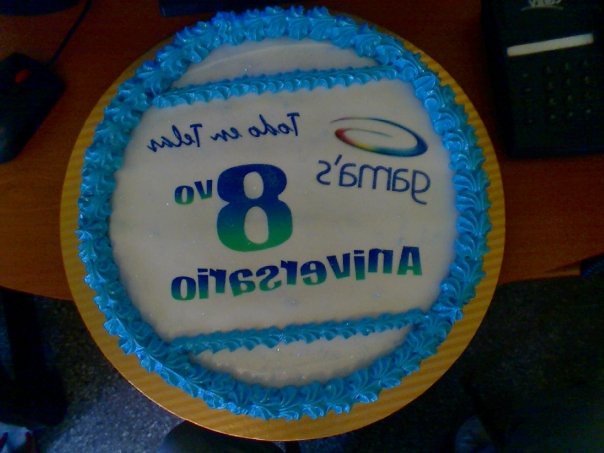The photograph features a single-layer white cake with blue icing accents, set on a round piece of cardboard. The blue icing forms a trim around the cake and two crossing lines on top, giving it a design reminiscent of a baseball. In the center of the cake is the number "8," symbolizing an eighth anniversary, with words written in blue and green icing beneath it. These words, written in Spanish, read "8VO ANIVERSARIO" in a mirrored fashion, indicative of being from South America. The cake also features a rainbow-colored "G," representing the company "Gammas." The image is somewhat dark and appears to be taken on a computer desk, as a black mouse and calculator are visible in the background. The photo is taken from an overhead perspective, highlighting the cake as the focal point despite its amateur quality.